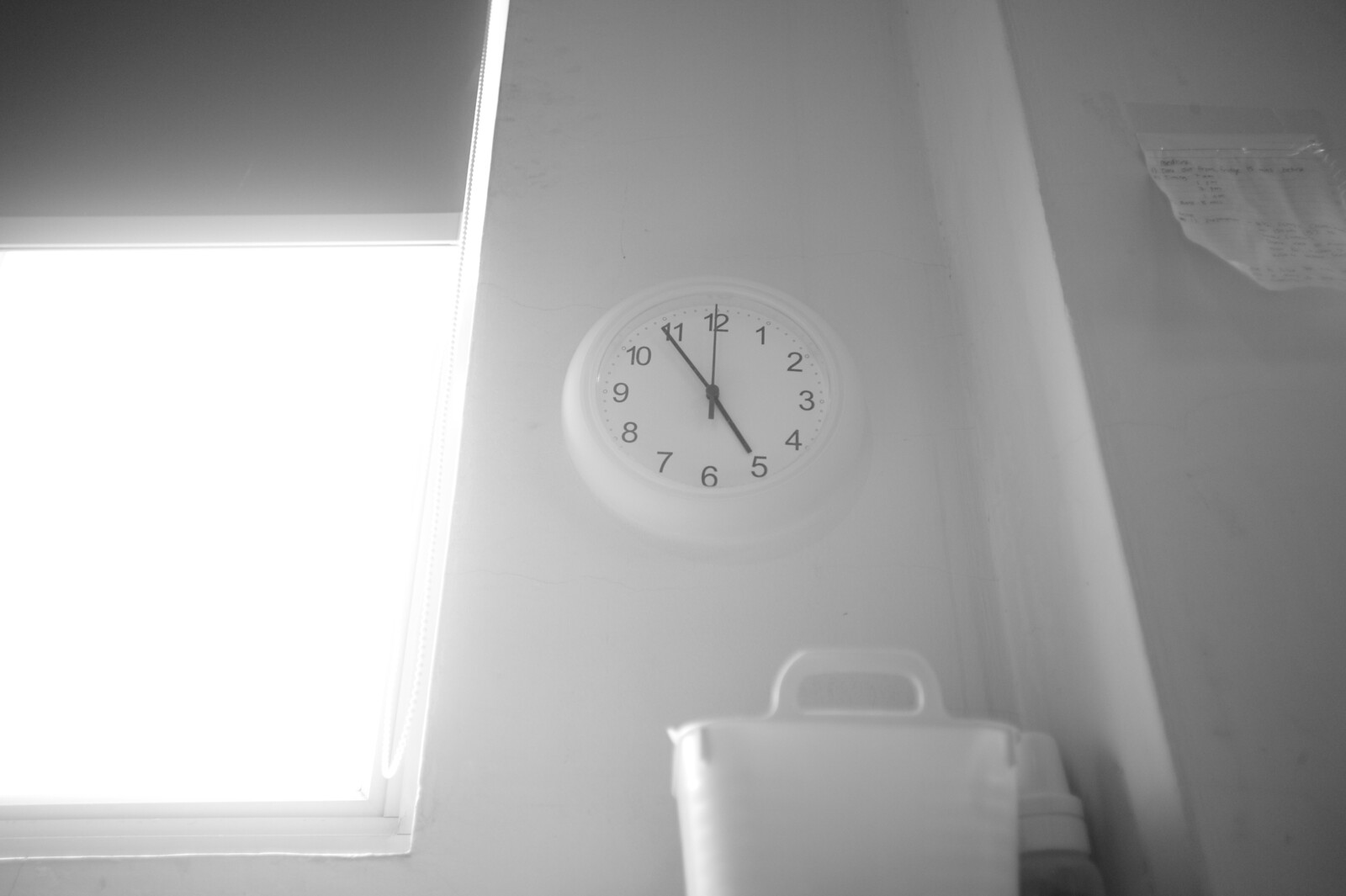This photograph depicts an overexposed room with predominantly white elements, contributing to its modern, monochromatic aesthetic. The white walls are interrupted on the left by a rectangular window framed in white wood, through which a deep, bright light filters, almost whitewashing the area. The window features a partially drawn blind, hanging about a third of the way down. Dominating the upper portion of the main wall is a circular clock with a white housing and face, adorned with black numbers, hash marks, and hands; the hour hand points to 5, the minute hand hovers near 11, and the second hand rests at 12, indicating it is approximately 5 minutes to 5.

Beneath the clock sits a white container with handles, likely a wastebasket or a small hamper. To its right, a piece of paper with black writing is taped to the wall at several points, adding context or perhaps serving as a list. The right side of the image features a white pipe extending from floor to ceiling, and nearby, an ambiguous cylindrical object tapers to dark gray at the base, suggesting it could be part of a shower fitting or another piece of plumbing. Shadows subtly shift the white walls to gray near the edges, enhancing the overexposed, high-contrast effect of the photograph, which may have been taken using modern black and white film.